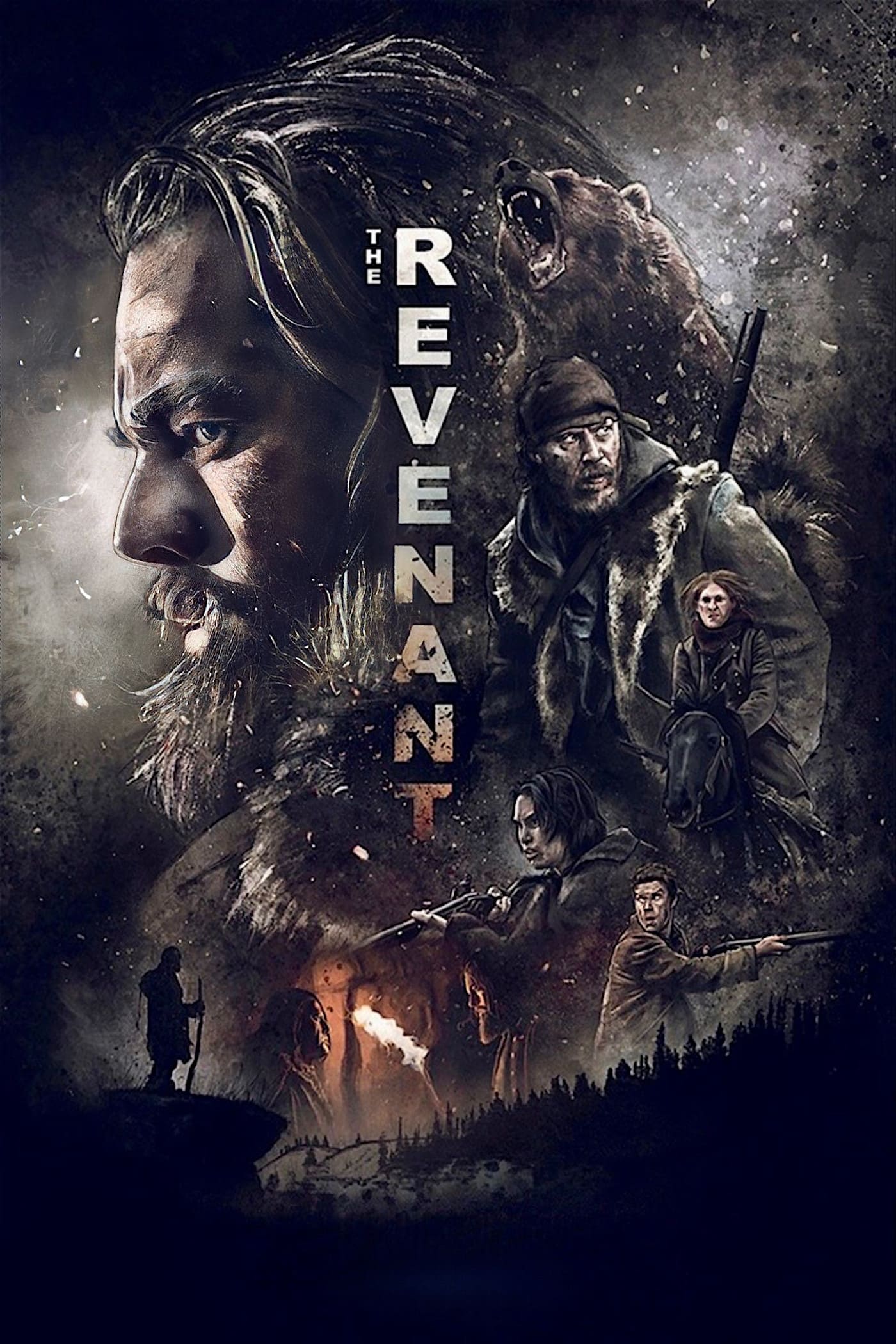The image is a poster for "The Revenant," rendered in a somber, dark palette dominated by black, brown, and gray hues. At the top, it features a large, zoomed-in side profile of a rugged outdoorsman, showcasing only the left side of his face. His stern expression, long hair, and full beard evoke a sense of raw survival and determination.

Descending vertically through the center of the poster is the movie's title, "The Revenant," which stands as a bold anchor between the various detailed elements within the artwork. Overlaying the main profile image are intricate and immersive illustrations that contribute to the gritty frontier theme. One drawing depicts a man clad in a fur coat with a rifle slung over his shoulder, gazing intently over his back. Another vivid element is a roaring grizzly bear, exuding a sense of wild danger. Additional characters populate the scene: a woman galloping on a horse, two figures aiming their rifles, and a group huddled in a cave, illuminated by the flicker of a torch. The backdrop is completed with the faint outline of towering trees, encapsulating the wilderness setting fundamental to the story.

The detailed composition and muted tones of the poster effectively convey the harsh, untamed world of "The Revenant," promising a gripping tale of survival and confrontation with nature's fiercest elements.